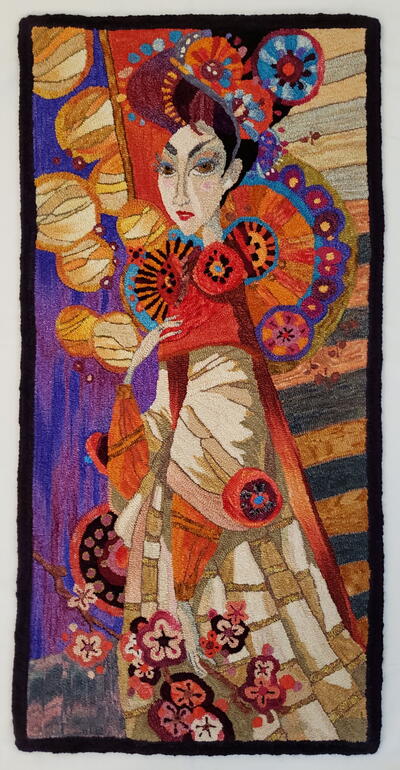This is a vertically aligned rectangular painting with a black border, set against a light gray background. The artwork is highly detailed, with intricate designs and a rich color palette that includes blues, oranges, yellows, brick reds, creams, tans, and pinks. The central figure in the painting is a woman who appears to be of Chinese descent. She is depicted in a side view, standing gracefully with her right arm raised to her chest.

The woman is adorned in a traditional, old-style gown that is predominantly red and cream-colored. The gown has a baggy, gold-colored section and features an array of floral patterns, especially towards the bottom. She wears a floral bonnet that complements her outfit and has her hair stylishly upswept. Her facial features are distinct, with a stern expression, pointy chin, blue eyeshadow, and dark upward-arching eyebrows.

To the left of the woman, the background appears to be an outdoor setting with vertical streaks of blue and purple, and some round-shaped, brown-colored objects that resemble bowls or possibly walnuts. On her right side, there are vertical strips of brown and blue colors. Towards the bottom left of the painting, there's an area colored in purple. The overall composition, including the colorful headdress and variety of fabric-like flower designs, suggests an elaborate and culturally rich depiction.